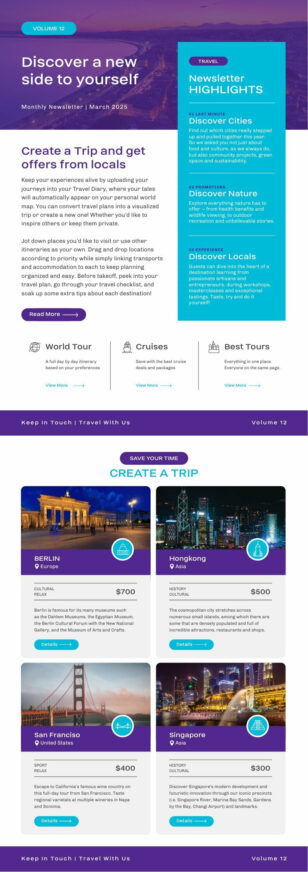Screenshot of a travel-focused website, viewed on a smartphone or tablet:

At the top, a blue oval button reads "Volume 12." On the right-hand side, a cyan rectangle contains a purple oval button with white text displaying "Travel." Below it, bold text states "Newsletter Highlights," followed by sections titled "Discover Cities," "Discover Nature," and "Discover Locals."

On the left side, a semi-transparent purplish rectangle overlays a cityscape, giving the water in the image a purple hue. At the bottom of this cityscape, white text reads "Monthly Newsletter," followed by a line and "March 2025."

In a white section below, bold purple text proclaims, "Create a trip and get offers from locals." Black text underneath explains the features: "Keep your experiences alive by uploading your journeys into your travel diary where your tales will automatically appear on your personal world map. You can convert travel plans into a visualized trip or create new. Whether you'd like to inspire others or keep them private, jot down places you'd like to visit or use others' itineraries as your own. Drag and drop locations according to priority, while syncing transports and accommodations to keep planning and organizing easy. Before takeoff, peek into your travel plan, go through your checklist, and search about each destination." (Parts of this text appear blurred due to zooming.)

A button labeled "Read More" with an arrow to the right is beneath this text. Further down, purple text states "World Tour Cruises" and "Best Tours."

At the bottom, a purple bezel reads "Keep in Touch" with a line and "Travel with us." On the right, another "Volume 12" label is seen beside an oval button with white text saying "Save Your Time" and cyan text urging "Create a Trip."

The site also showcases various cities: an image of Berlin with its name below, a skyline of Hong Kong with black and blue skyscrapers, the Golden Gate Bridge labeled "San Francisco," and a cityscape of Singapore featuring yellow, green, and purple-lit skyscrapers.